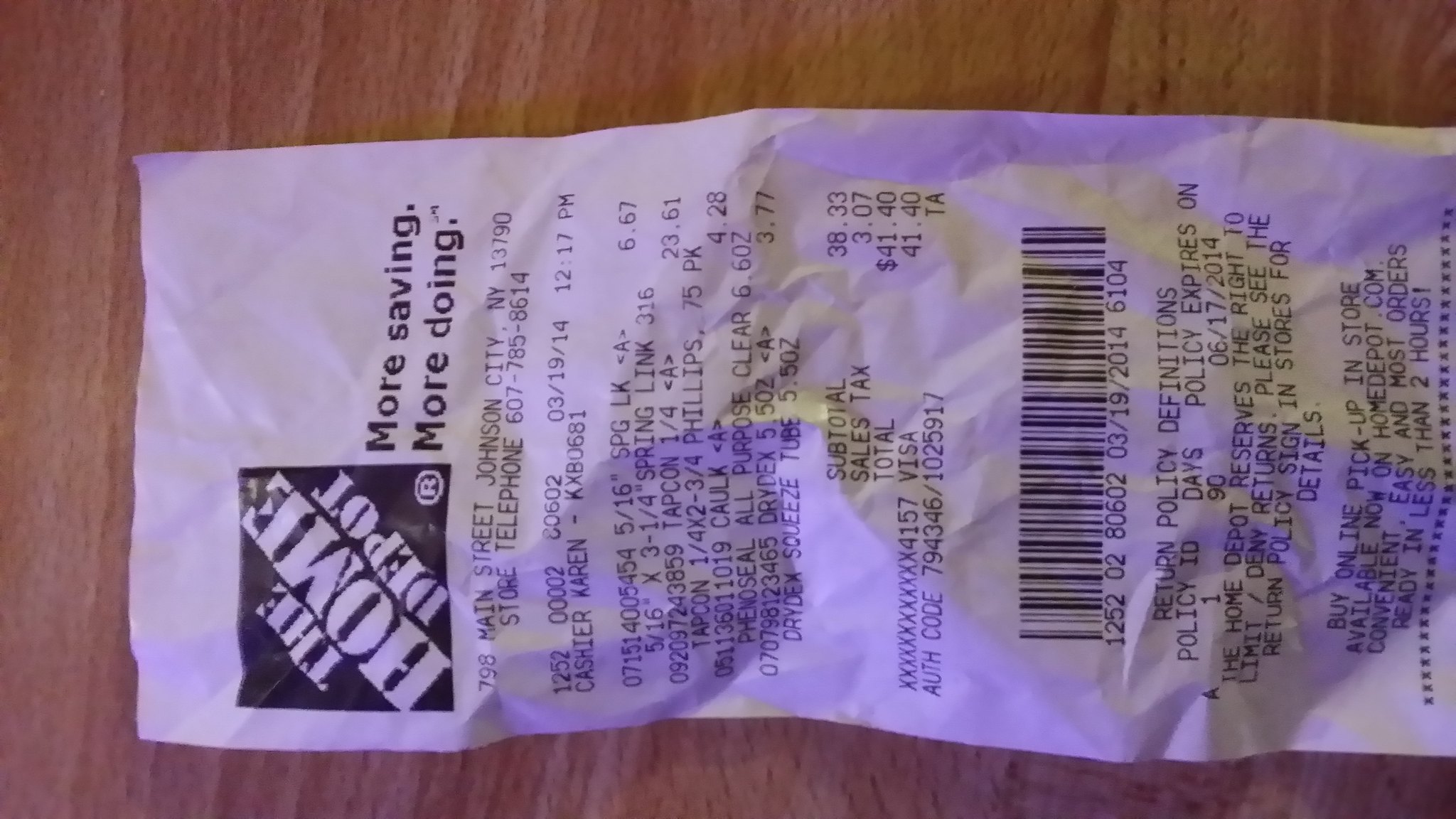This detailed photograph showcases a Home Depot receipt resting on a medium brown, textured wooden surface. The receipt, slightly crinkled, displays "The Home Depot" logo prominently at the top left corner within a black box, accompanied by the slogan "More Saving. More Doing." It is from the Johnson City, New York store, located at 798 Main Street, with a purchase made on March 19th, 2014, at 12:17 PM. The cashier on duty was Karen. The total amount of the purchase was $41.40, paid via Visa, and the receipt features a UPC barcode at the bottom.

The items purchased include a 5 16ths by 3 quarters spring link, a 75-pack of Tapcon 1 quarter by 2 and 3 quarter Phillips screws, Fano seal all-purpose clear caulk, and a Drydex squeeze tube, likely another caulking product. The detailed transaction is evidenced by typical black lettering on a standard white receipt, highlighting the specifics of each item and their respective prices: the Phillips screws pack at $23.61, the all-purpose clear caulk at $4.28, and the Drydex squeeze tube at $3.99.